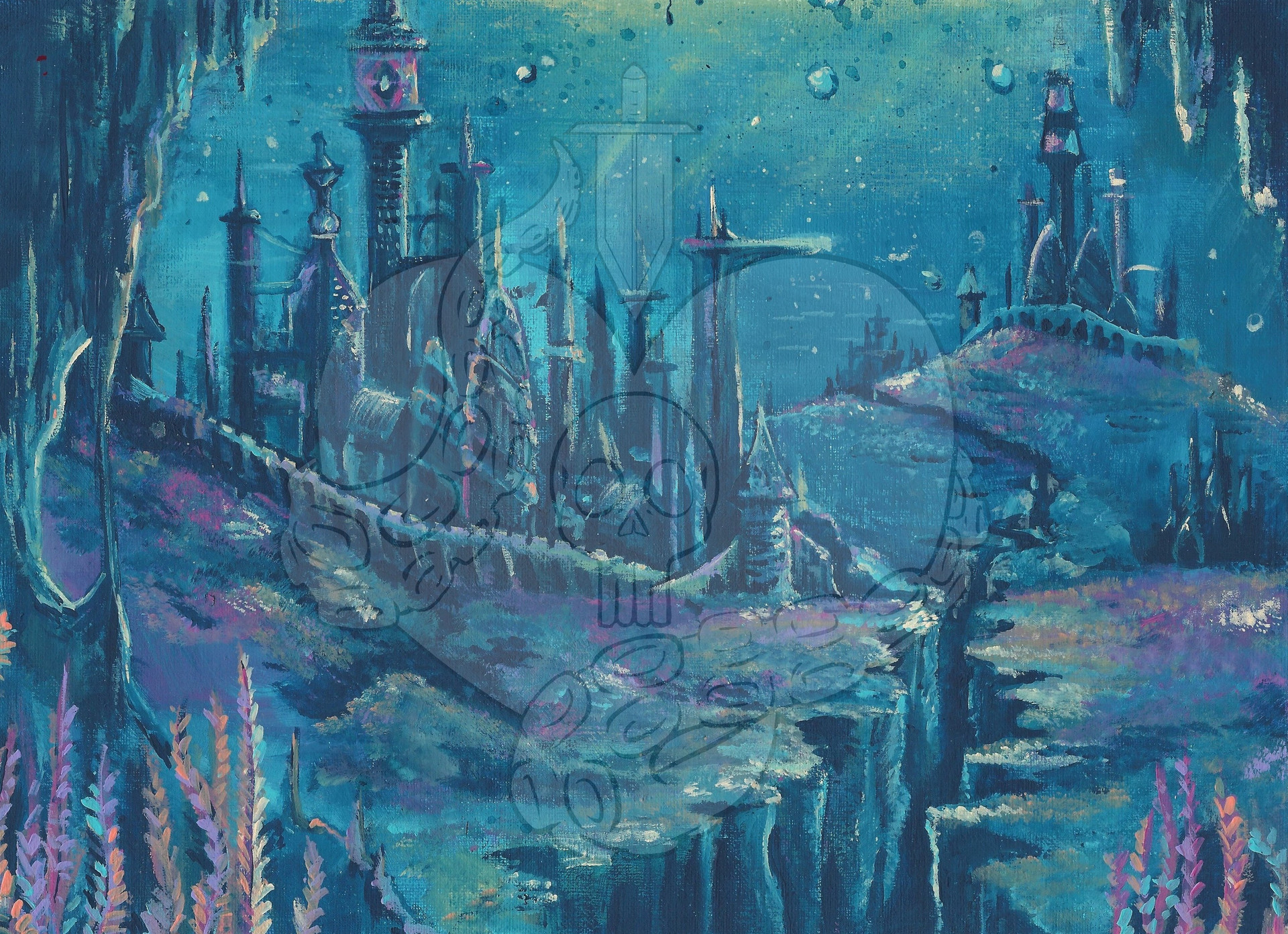The image depicts a fantastical underwater city, presented either through a painting or a digitally created artwork, set in shades of teal, pink, and muted purples. The composition is horizontally oriented, resembling a scene from a fantasy novel or a sci-fi realm with an aquatic ambiance. The foreground features cave-like elements with stalagmites and stalactites, and a ravine running through the ground, creating a vibe of a submerged cavern. Delicate pink, yellow, and peach-colored plants grow from the bottom on both sides, adding vibrant touches to the mystical environment.

In the mid-ground, a faint watermark depicts a heart entwined with a skull, an octopus tentacle, and a knife, subtly blending into the scene. Scattered bubbles and a soft blue light contribute to the underwater or foggy appearance, enhancing the surreal atmosphere.

Further back, there are structures that faintly resemble castles, with steeples and spires illuminated by distant lights, giving an impression of an expansive underwater kingdom. One prominent castle-like structure stands on an underwater hill to the left, with another counterpart to the right, and a third further back, creating depth and a sense of a sprawling realm. The cityscape and flora lend an eerie, other-worldly charm to the image, reminiscent of a fairytale night scene without any inhabitants, only mysterious and silent underwater architecture and botanical life.